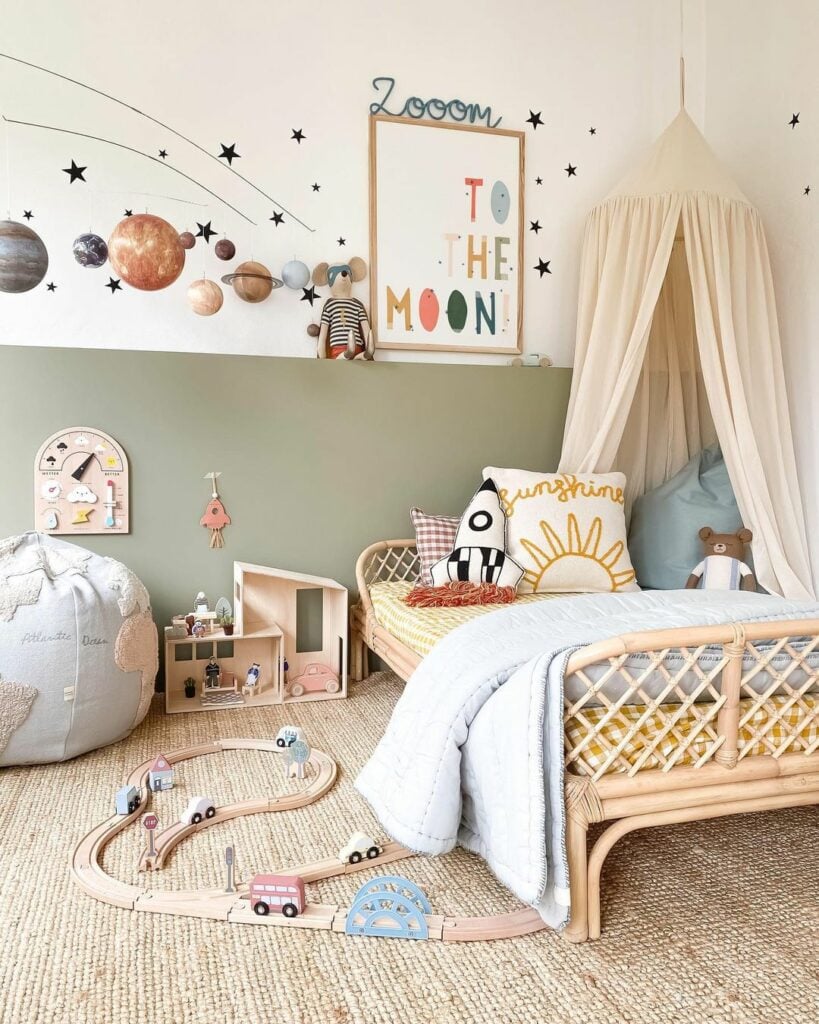The photograph captures a child's enchanting and well-decorated bedroom. The room features a short twin bed with a rustic, bamboo-like wooden frame adorned with various pillows, including ones shaped like a rocket ship and a sunshine, and a cuddly teddy bear in the middle. A whimsical canopy, possibly illuminated and made of sheer fabric, drapes over the bed, providing a cozy, sheltered nook. The carpeted floor beneath the bed resembles wicked wood and hosts an intricate wooden train set, complete with tracks, bridges, and miniature wooden trains and vehicles. To the right of the bed, there's a playful dollhouse and a plush beanbag chair that resembles a globe, embroidered with the continents. The walls are a celestial canvas, painted with vibrant planets from our solar system and sprinkled with black stars, complemented by a motivational poster proclaiming "Zoom to the Moon."